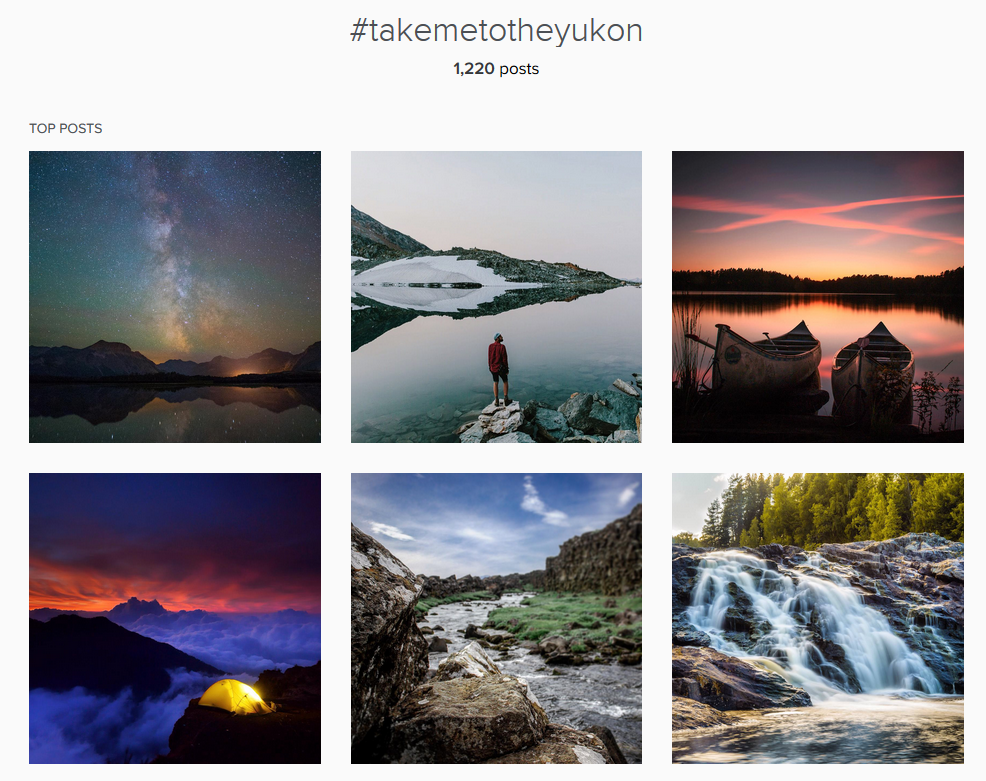The image appears to be a meticulously arranged web screenshot featuring a collage of six captivating outdoor scenes, presented against a very light gray, almost white background. The collage is divided into two rows with three photos each, creating a visually pleasing symmetry.

At the center top of the image, black text prominently displays the hashtag "#TakeMeToTheYukon". Below the hashtag, the number "1,220 posts" is noted, suggesting the popularity of this theme. The label "Top Post" is situated in the upper left-hand corner, marking the significance of the collection.

1. **Top Left Photo:** A breathtaking nighttime shot where the Milky Way arcs majestically across the sky, framed by rugged mountains and a tranquil body of water. The ethereal beauty of the Milky Way is the focal point, drawing the eye to the center of the image.

2. **Top Middle Photo:** Capturing the serene moment of either dusk or dawn, this picture shows a solitary person standing on a rock by a lake. Surrounded by mountains on the left and a gray sky, the person gazes at their reflection in the still water. A bridge or another rock-like formation adds interest to the scene.

3. **Top Right Photo:** This pre-dawn or post-dusk image features a dramatic sky where dark blue at the top graduates into red-hued clouds and a subtle yellow glow near the horizon. Mountains silhouette against the transitioning sky, and a few boats rest idly on the mirrored lake surface.

4. **Bottom Left Photo:** Depicts waves crashing onto mountain bases under a stormy, gray-blue sky. In the lower right corner, an inviting yellow glow emanates from a small, illuminated tent, suggesting the presence of a lone camper amidst wild nature.

5. **Bottom Middle Photo:** A scenic riverbank stretches between mountain ranges under a partly cloudy, blue sky. The gray waters of the river reflect the overcast mood of the scene, combining tranquility with rugged natural beauty.

6. **Bottom Right Photo:** A powerful waterfall cascades down, flanked by lush vegetation. Trees crown the waterfall's summit, framed by a gray sky in the upper left corner, capturing nature's relentless force and serene greenery in harmony.

This visually rich collage encapsulates the diverse and stunning landscapes of the Yukon, inviting viewers to immerse themselves in its rugged beauty and tranquil moments.